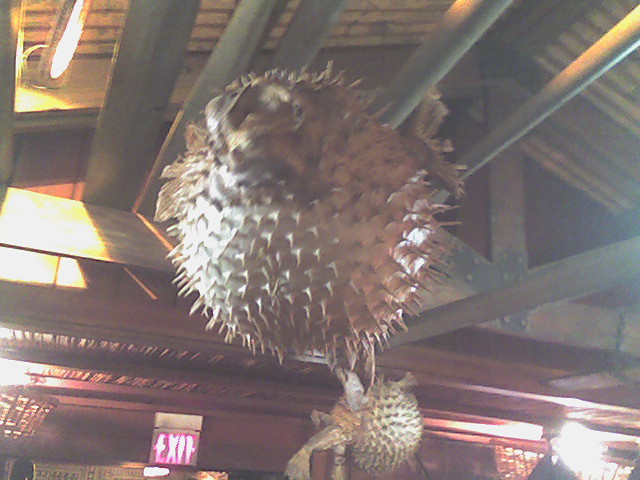The photograph captures the interior of a building, featuring a focal sculpture of an inflated blowfish-like object suspended from the ceiling. The ceiling is detailed with faded green rafters, a dimly lit corrugated roof, and wooden support beams. The primary blowfish is prominently centered, characterized by its light brown, spherical body, and sharp, brown spikes. It has a distinguishable face looking straight ahead. In the background, a smaller, similarly spiked object, which appears red, is also suspended, suggesting a thematic display. The left side of the image is illuminated, casting light onto a dark mahogany-red wall adorned with an exit sign. The scene blends the intricate, spiky sculptures with the structural elements of the building, creating a visually captivating indoor display.